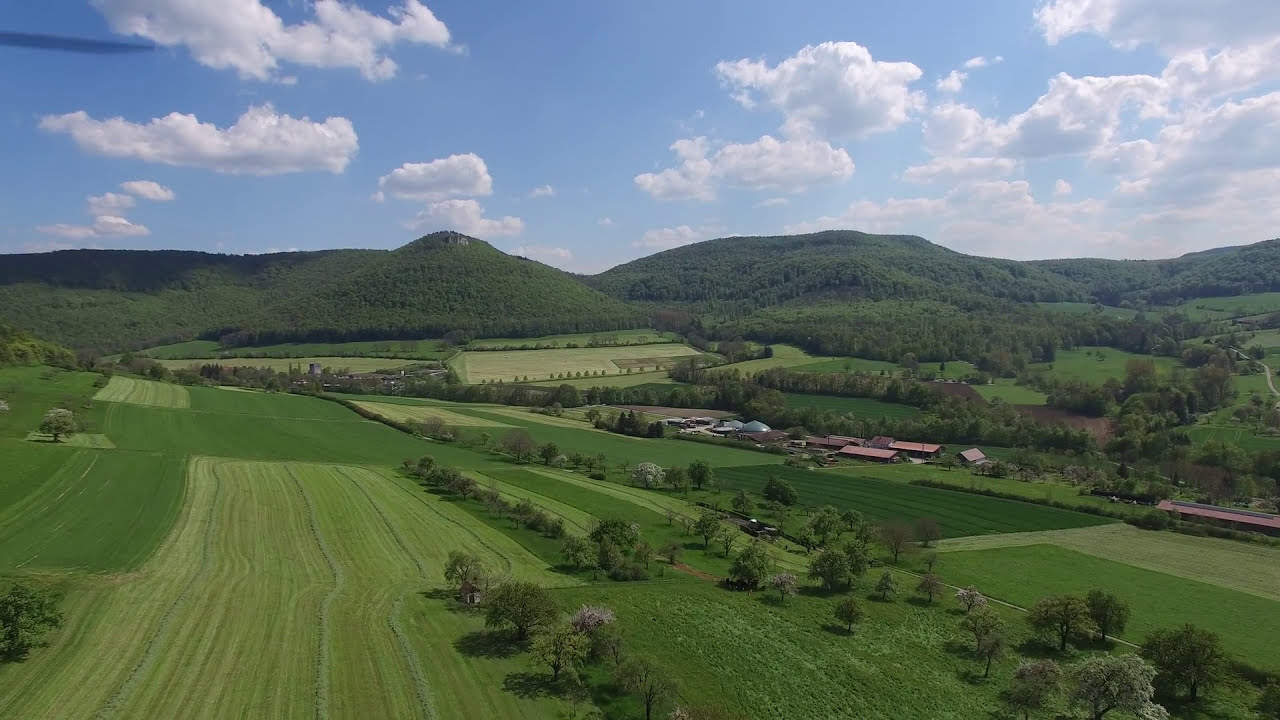The image depicts a vast expanse of meticulously cultivated farmland, characterized by neatly arranged fields that create a patchwork of various shades of green. Some fields are light green, while others are a darker hue, indicating different types of crops or stages of growth. Interspersed between these fields are irregular lines of trees with lush green leaves. Towards the center-right of the image, a cluster of small, single-story buildings is visible, featuring brownish-red roofs, likely indicating a farming community or village. Beyond the immediate farmland, the landscape transitions into rolling green fields and eventually rises into densely forested hills or mountains. The background hills are richly covered in greenery, with shadows cast by clouds adding depth to the scene. The sky above is a vibrant blue, dotted with numerous fluffy white clouds, suggesting a day with good weather.